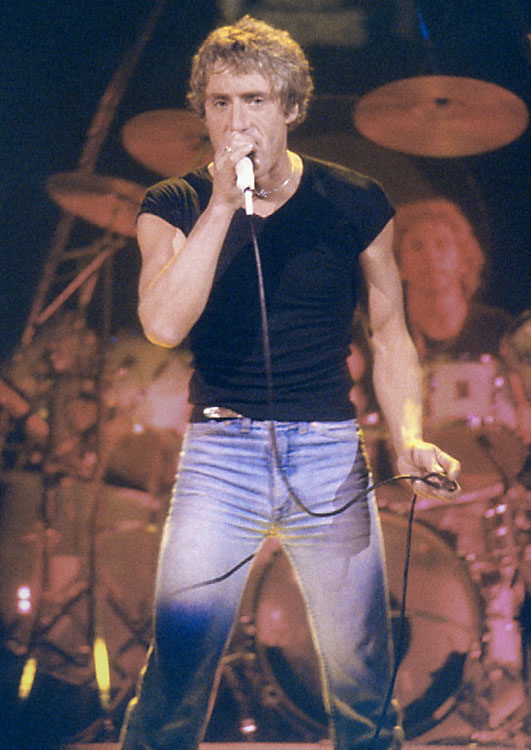This vintage, grainy photograph captures an electrifying moment at a concert. A spotlight illuminates the center-stage main performer, a man with short blonde hair and a muscular build, clad in a tight black short-sleeved t-shirt and skinny blue jeans. A silver necklace gleams around his neck as he passionately sings into a white microphone held in his right hand while gripping the mic wire with his left. Surrounding him, the stage is bathed in a vibrant red overlay that tints everything, including the drummer behind a sprawling drum set, blending elements into the crimson-toned background. The stage, set against an inky black sky, features various instruments and structures partially obscured by the dramatic lighting, drawing all focus to the animated singer in full color.